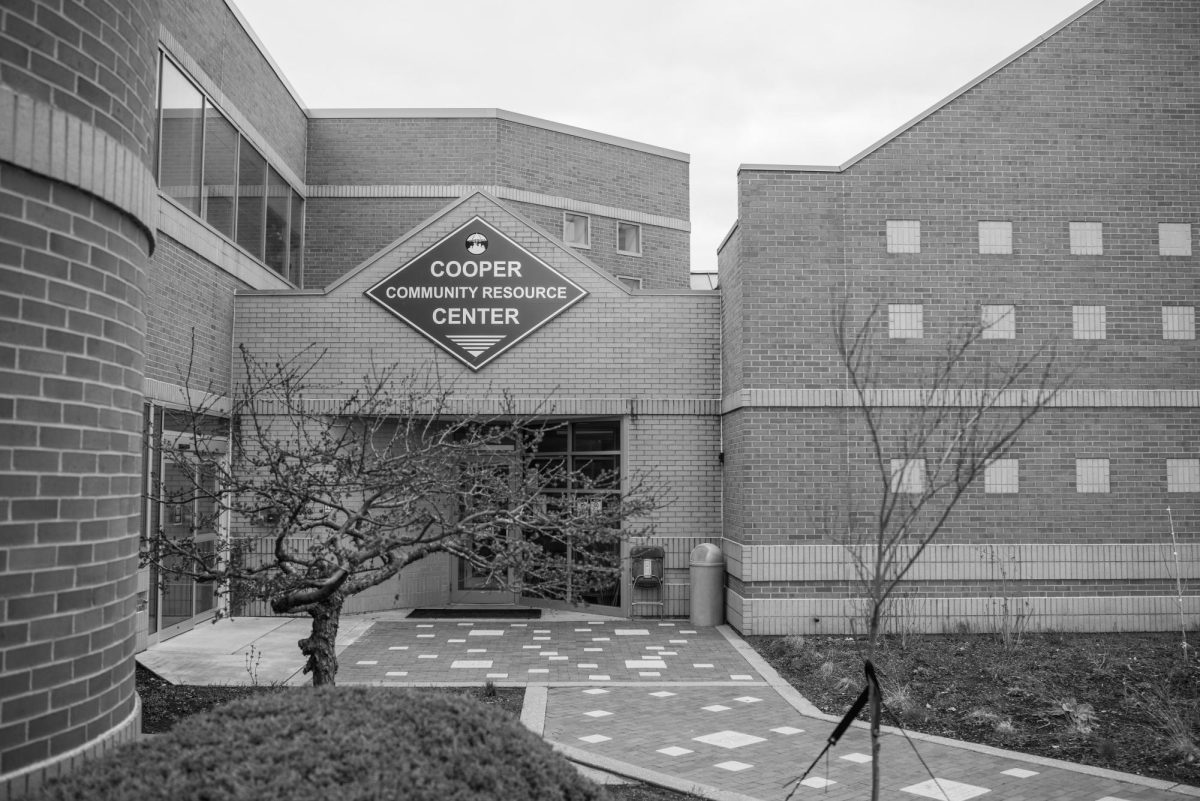The black-and-white photograph depicts a large, recently constructed brick building identified as the Cooper Community Resource Center, indicated by a diamond-shaped sign with a dark background and light letters. The building features a brick walkway leading to glass doors framed by a triangular brick motif above them. The structure appears to be two stories high, with several glass windows visible on the upper floor. The exterior is surrounded by a mix of dead-looking grass, shrunken plants, and saplings, with one tree showing faint buds. A gray trash can is positioned to the right of the entrance, and the landscaping includes mulch beds with shrubs and small trees supported by stakes. The sky is overcast, contributing to the photo's overall wintry, desolate atmosphere.